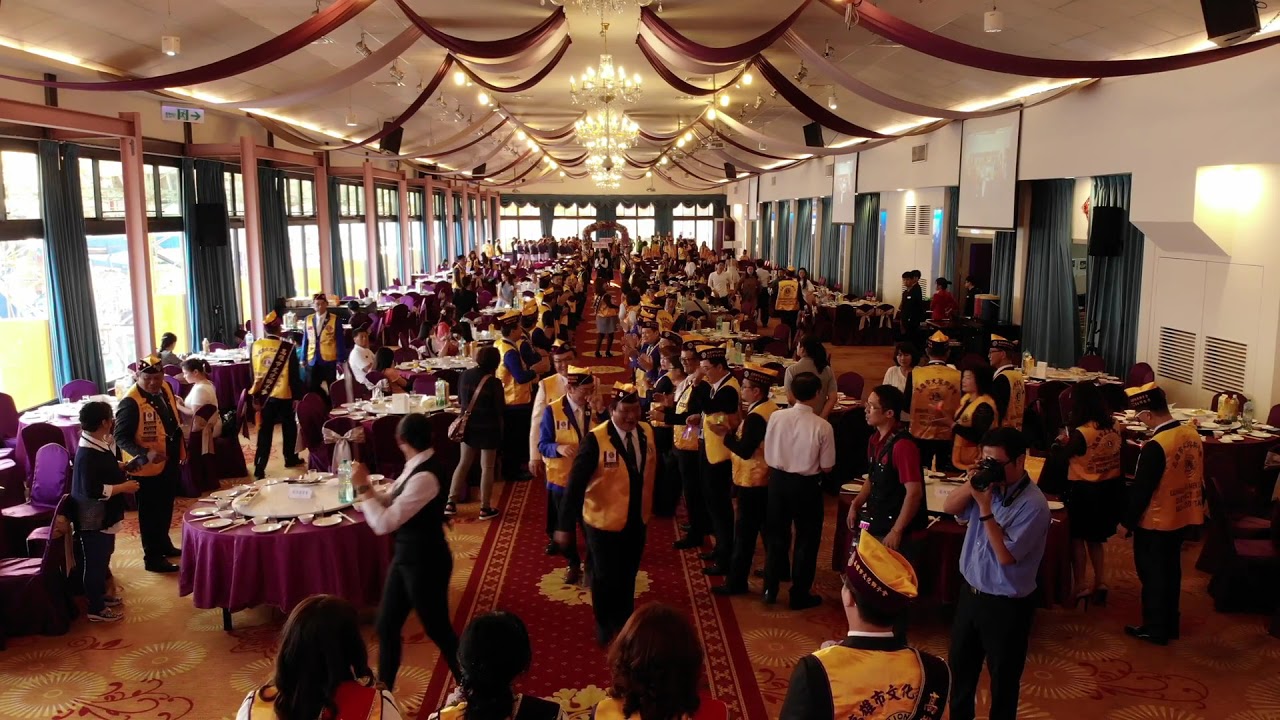The image captures a vibrant banquet hall scene from above, showcasing a festive event. The long hall features pristine white walls on one side, with tall windows draped in elegant green curtains along the end and left side. The ceiling, adorned with alternating maroon and pink banners, highlights at least one central glass chandelier, flanked by other lighting fixtures. Greenish curtains partition doorways leading to areas like the kitchen or coat room. The floor is covered in a vivid floral-patterned carpet in shades of red, yellow, and orange.

The room is bustling with guests seated at circular tables, arranged in four rows, covered with purple tablecloths and set with white place settings. Dozens of attendees are dressed in distinctive attire: shiny yellow vests over black pants and long-sleeved shirts, topped with matching yellow hats, reminiscent of a military or pseudo-military style, possibly similar to Shriners. Some guests wear dark sashes, and everyone is engaged in various activities—chatting, drinking, or posing for pictures. Interspersed among the guests, waitstaff can be identified by their white shirts and black vests, moving efficiently through the event. A red carpet walkway adds to the festive atmosphere, guiding guests through this lively and meticulously decorated banquet hall.